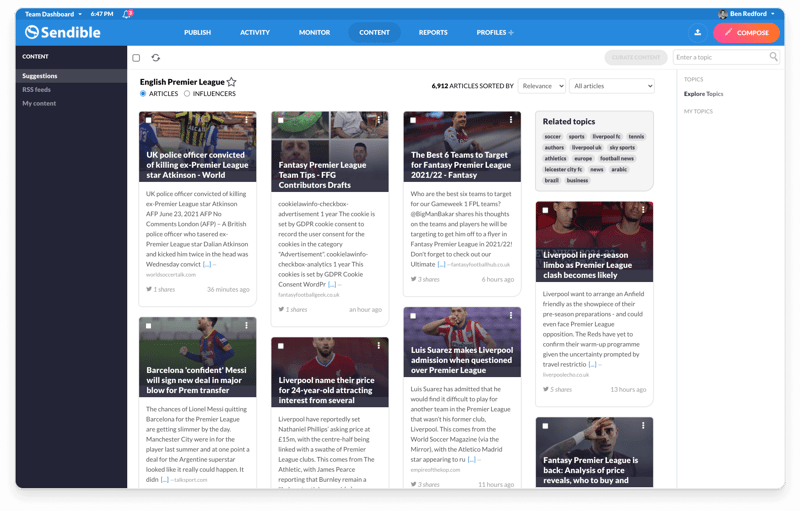A screenshot of the Sendable platform prominently displays its name in the upper left-hand corner, accompanied by a partially obscured icon resembling a globe. Above this, in small text, it reads "Team Dashboard" and the time "8:47 PM" or possibly "6:47 PM." In the upper right-hand corner of the screenshot, a notification bell is visible along with the user name "Ben Bredford," elements that appear to be from the user's desktop rather than the Sendable platform itself. The main content area of Sendable showcases numerous articles related to sports, specifically soccer (football in many countries). The left-hand side features a menu, with the "Content" section visible and "Suggestions" highlighted, indicating the active selection. Below this are options for "RSS Feeds" and "My Content." The header highlights articles pertaining to the English Premier League, reaffirming the soccer theme.